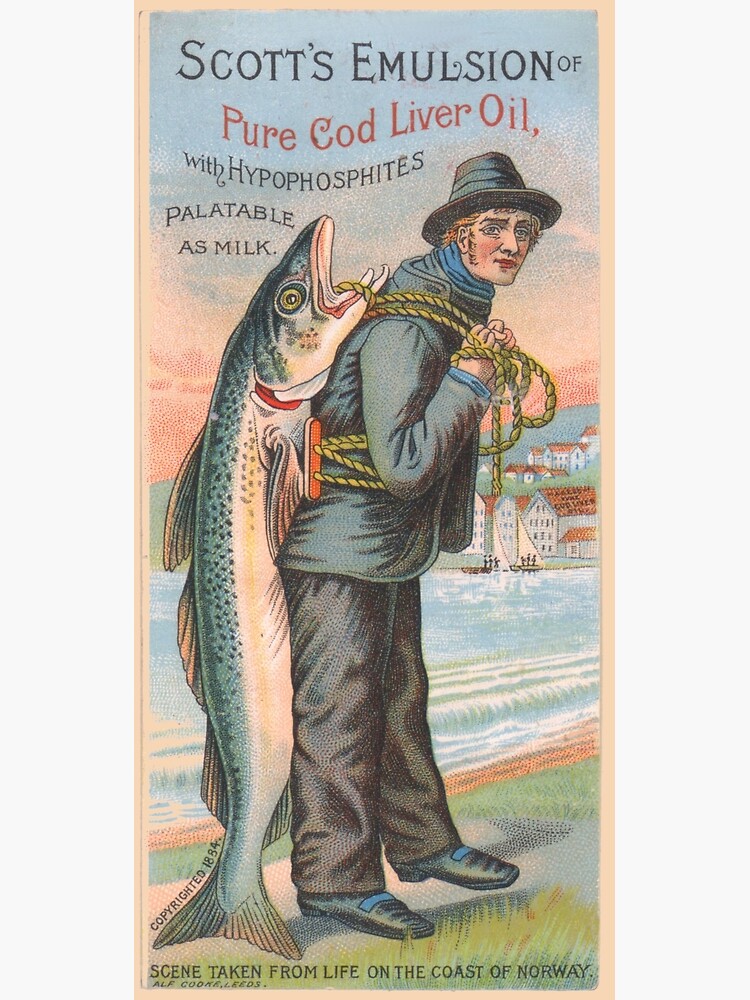This captivating vintage advertisement from 1884 depicts a robust man wearing a black suit, hat, and shoes, leaning forward with a massive codfish strapped to his back. The fish, illustrated in colored pencil with ink outlines, stretches from his head down to the ground, nearly matching his height. The man is positioned in profile, facing right, and stands on a grassy bank in front of an ocean. In the distance, charmingly drawn houses dot a hillside, and people can be seen along the shore. At the top of the ad, bold lettering announces, "Scott's Emulsion of Pure Cod Liver Oil with Hypo Phosphites Palatable as Milk." At the bottom, in much smaller font, it reads, "Scene taken from life on the coast of Norway," accompanied by a copyright notice dating back to 1884, confirming its 19th-century origin.